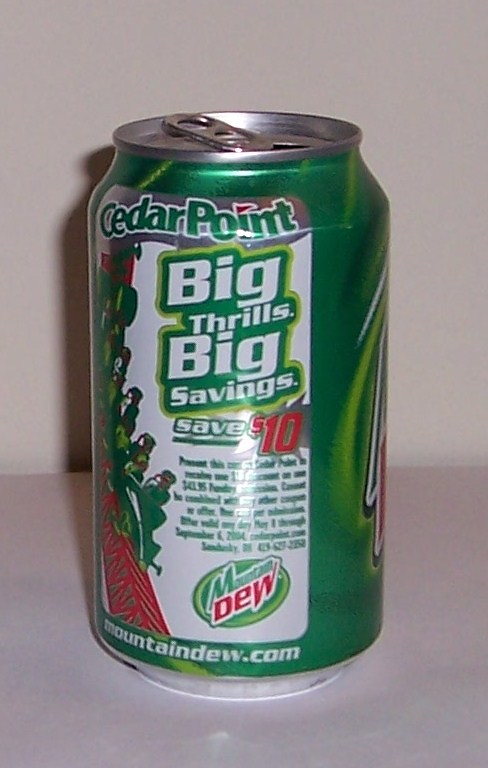This is a detailed descriptive caption for the given photograph:

"A photograph showcasing an open aluminum can of Mountain Dew. The can is positioned with its front label turned away, prominently displaying an advertisement on its backside. The ad reads 'Cedar Point - Big Thrills, Big Savings, Save $10,' featuring a green roller coaster cartoon with riders descending a red track to the left side. Below the advertisement, the Mountain Dew logo is visible, and at the bottom, the URL 'MountainDew.com' is printed. The can rests on a gray table with the light source illuminating from the bottom right, casting a shadow behind and to the left of the can. An off-white wall serves as the backdrop, enhancing the focus on the can."